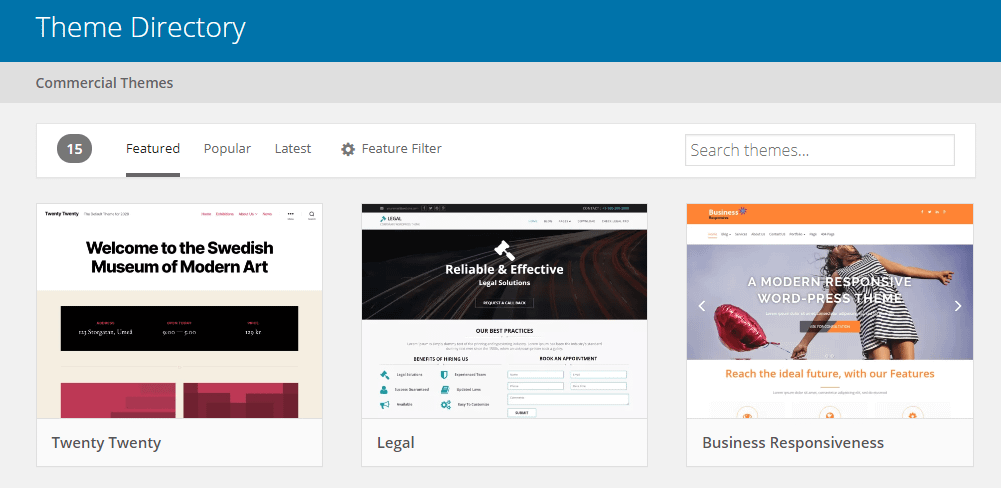The image features the theme directory of a website, displaying various highlighted sections and options for choosing themes. At the very top, there is a sleek, blue rectangular navigation bar, with "Commercial Themes" prominently displayed within a grey rectangle also at the top. Just below this, a grey circular icon with the number "15" leads, followed by the word "Featured" underlined, indicating a selected category. The options "Popular," "Latest," and "Feature Filter" are aligned horizontally next to it. In the bottom right corner of this section, there's a search bar labeled "Search themes..."

Further down, the directory exhibits three distinct theme boxes aligned horizontally. The left box promotes the "Swedish Museum of Modern Art" with "2020" inscribed at the bottom. The center box features the terms "Reliable and Effective" and "Legal." The right box showcases a "Modern Responsive WordPress Theme" and includes the labels "Business" and "Responsive," along with a hint of orange highlighting certain elements.